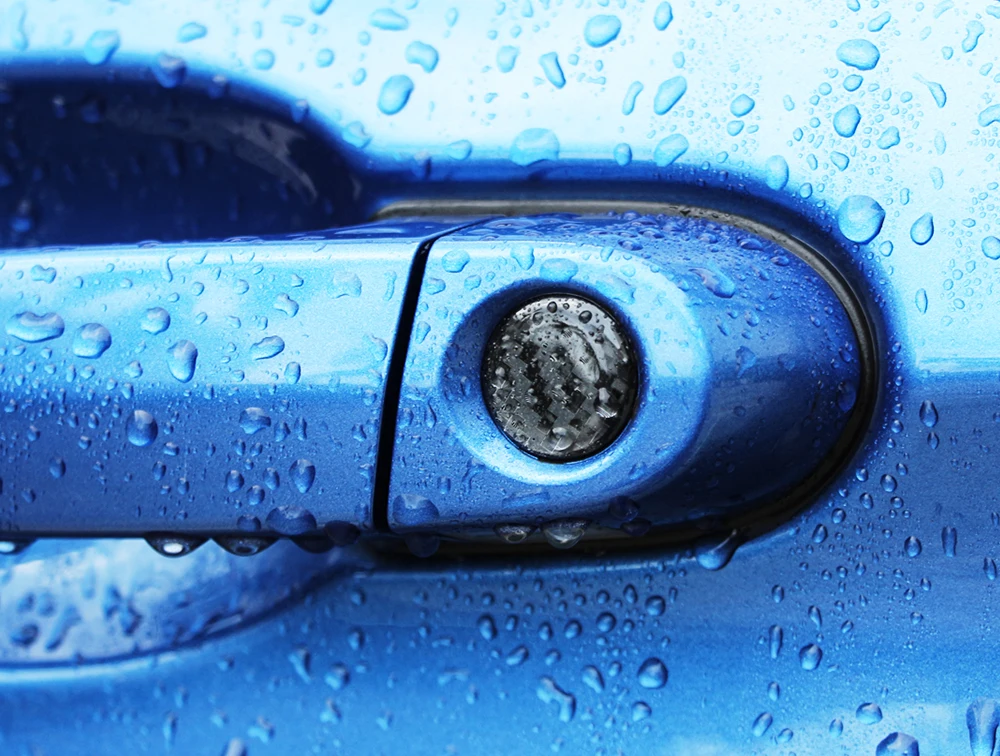This is a highly detailed, close-up photograph of a car door handle in the rain. The car is painted a striking shade of blue, with the hue appearing darker at the bottom and gradually becoming lighter towards the top. The handle casts a shadow on the lower part of the door. Above the handle, the surface is illuminated, highlighting the smooth, glossy finish of the waxed surface. The handle indentation, where one places their hand to open the door, is clearly visible. On the right side of the handle, there is a black push button used for locking the door. The car door is covered in water droplets, some large and stationary, others smaller and trickling down, emphasizing the wet conditions. The handle itself is positioned towards the left side of the horizontal, rectangular image, contributing to the composition's balanced yet dynamic feel.